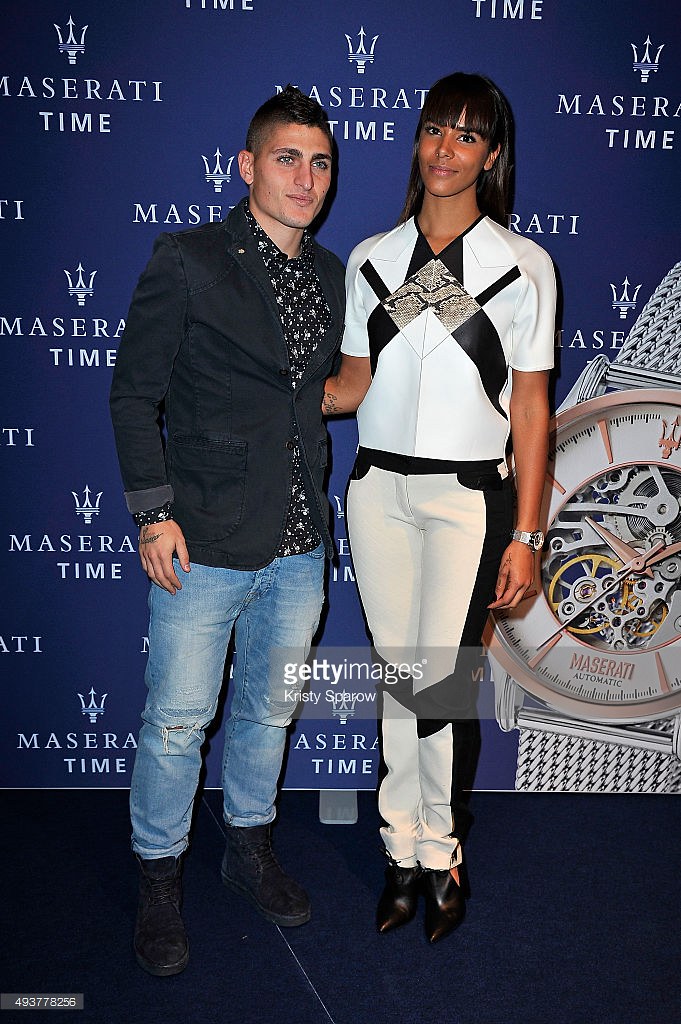In this vibrant, color-filled image, a well-dressed gentleman and a stylish woman are capturing a moment at what appears to be a promotional event. The gentleman, of lighter skin complexion, sports a sleek dark suit paired with blue jeans, dark boots, and a scarf, while the woman, of darker skin complexion, is elegantly attired in a white outfit accented with black trim, which extends from her top down to her dark shoes. They stand close together, smiling and looking directly at the camera. The backdrop features a dark blue wall adorned with repeated "Maserati Time" logos and an image of a silver watch labeled "Maserati Automatic." The scene is brightly lit with natural light, highlighting the clear and lively setting. Visible in the bottom left corner of the image, there's a long number, 493778256. This photo, marked with a Getty Images watermark and credited to photographer Christy Sparrow, exudes an aura of sophistication, suggesting that it captures a moment at an exclusive event.